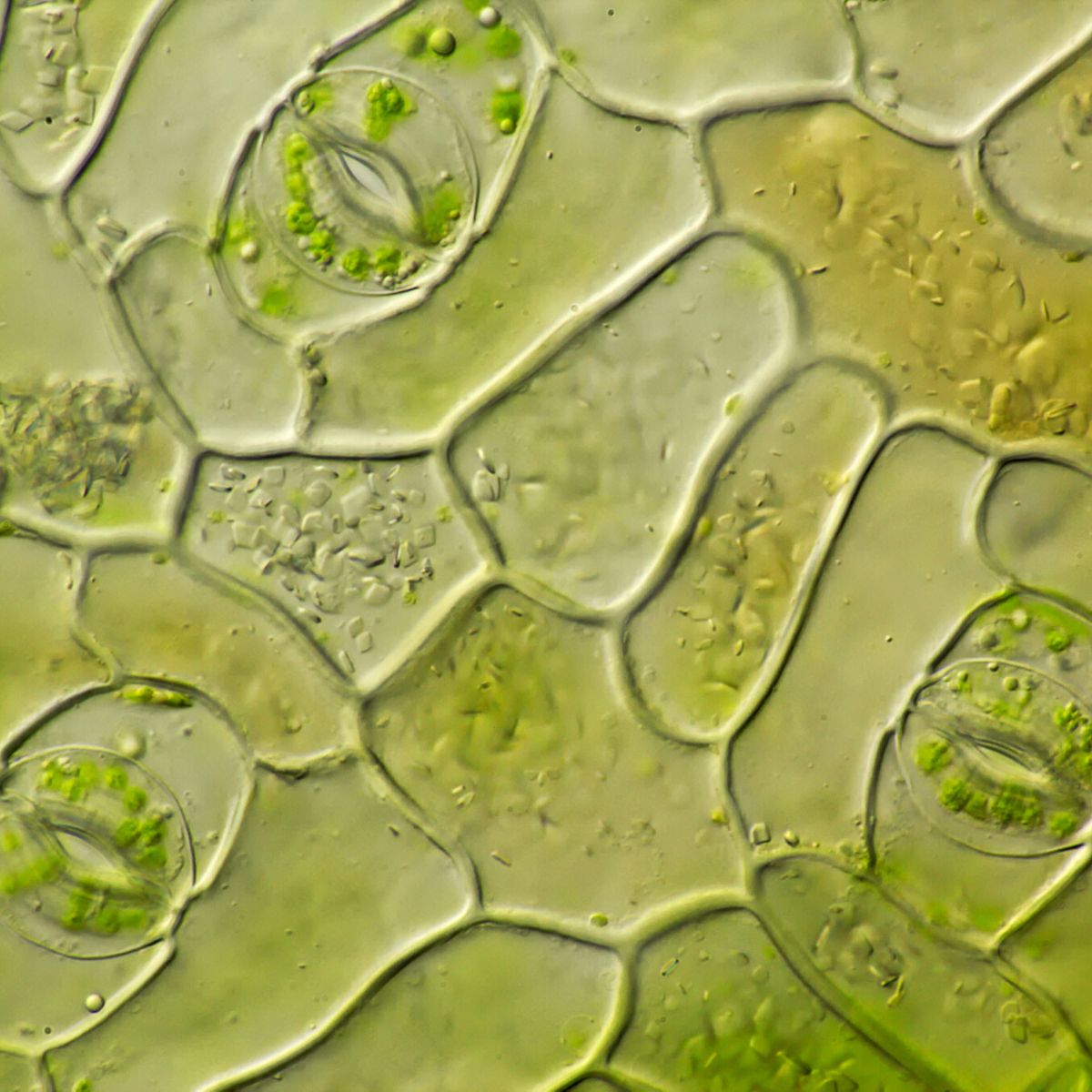The image is a highly detailed microscopic photograph of an organic material, predominantly showcasing varying shades of green, including lime green, against a backdrop of black and gray. The scene depicts a textured, waxy surface accentuated by ridges and upraised borders that create irregular, bean-like shapes. Scattered across the surface are three distinct, eye-shaped objects, with one positioned at the top left, another at the bottom left, and the last one at the bottom right. These intriguing eye-shaped features seem to integrate seamlessly with the overall skin-like texture, adding a unique aspect to the already complex and intriguing visual tapestry of this microscopic world.